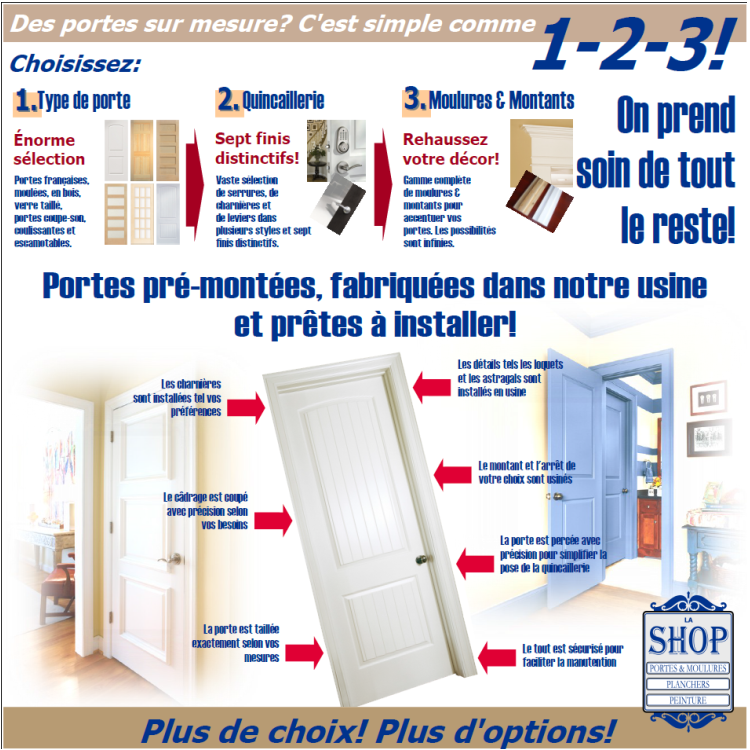This image is an advertisement for a company that sells doors, all written in French. The poster is richly detailed and designed in a modern, informational style with beige-colored stripes at the top and bottom, and dark blue sans-serif typography. 

In the top left corner, there are images showcasing various door styles and colors: a white door, a wood-colored door, and multiple shades ranging from light tan to golden and beech wood. Some of these doors feature windows. The second image prominently displays a doorknob on a white door. The third image highlights a piece of white crown molding above a doorway. 

In the center, there's an image of a crooked, tilted white door balancing on one corner, with arrows pointing to various features, emphasizing the customizability of the product. 

The bottom left of the poster shows a white door with three rectangular panels, partially open, revealing light streaming in from another room. 

In the bottom right corner, there is a blue door with a matching blue frame and two square designs. 

A blue sign for the shop, which says "La Shoppe," lists three types of merchandise they sell, with scroll motifs framing top and bottom, and the banner below reads, "Plus des choix, plus des options" (More choices, more options). This ad clearly illustrates the variety of doors, handles, and crown moldings available, inviting customers to customize their selections.